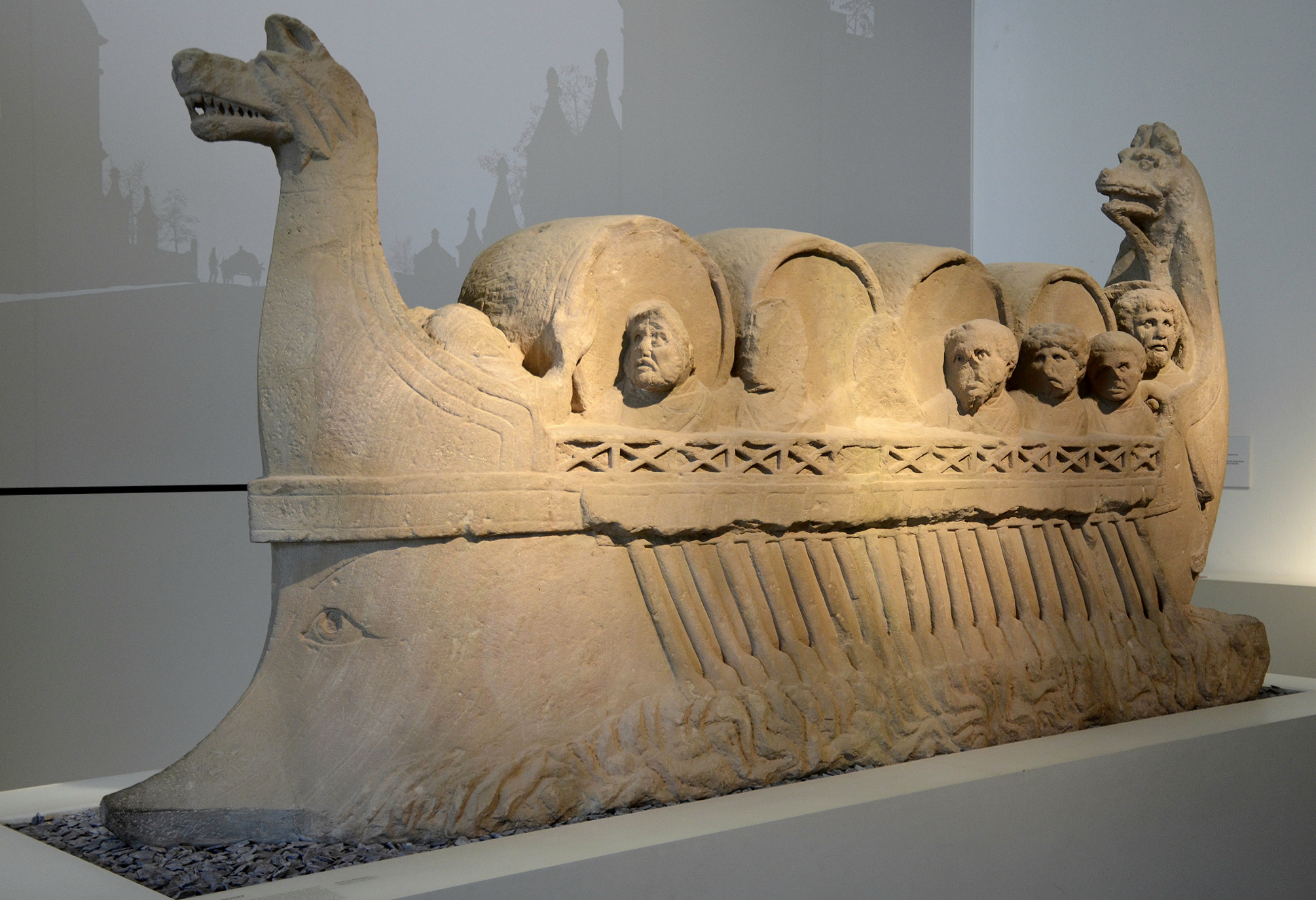The image depicts a detailed stone artifact displayed in a museum, characterized by white floors, white walls, and soft lighting which highlights the piece. This ancient, brown-hued stone sculpture resembles a Viking ship or potentially even an older type of vessel. The ship is ornate, featuring intricately carved animal heads, possibly dogs, jackals, or horses, adorning both the bow and stern. Along the interior, the artifact showcases reliefs of seven people, some worn or damaged, each appearing to support barrels on their shoulders. Despite the evident wear, the sixth and seventh figures retain significant detail. The artifact rests on a white base, surrounded by plain white walls, amidst a setting potentially featuring some subtle shadowy imagery of buildings in the background. The meticulous detailing and museum presentation underscore its historical significance.